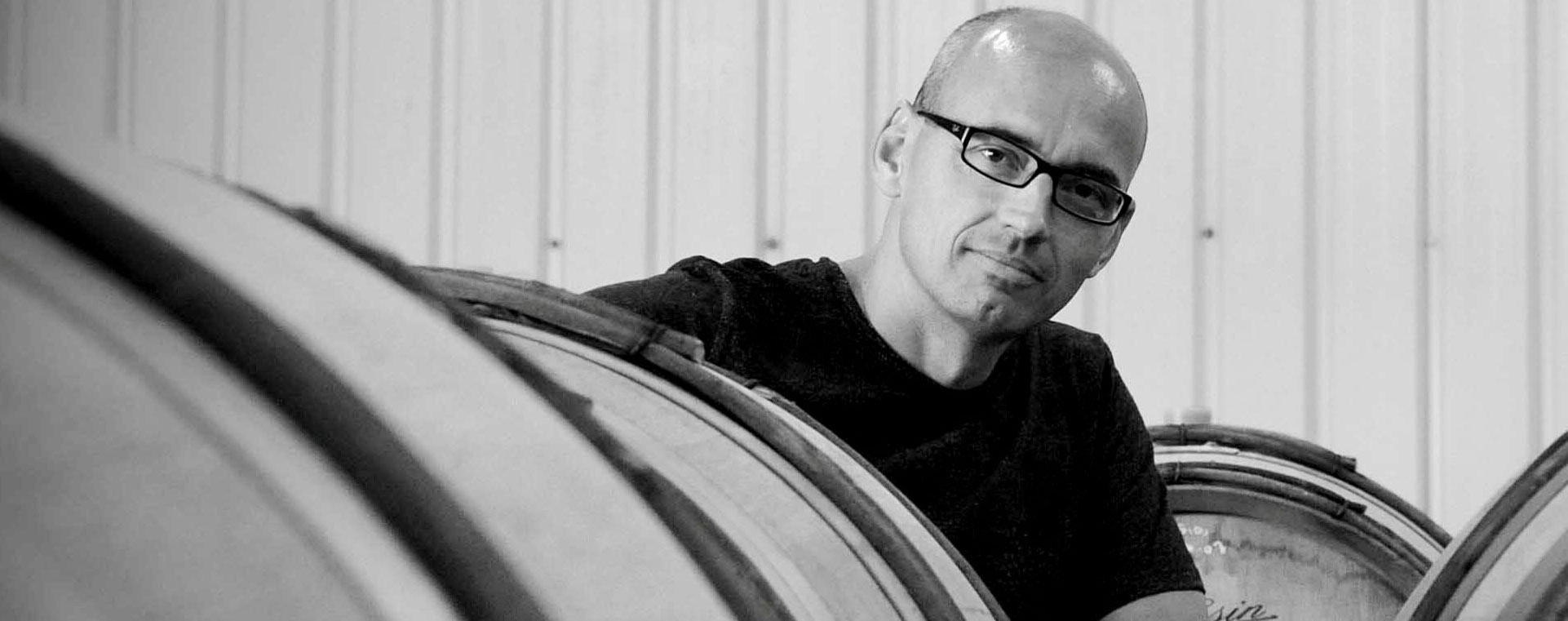In this black-and-white photograph, a bald, clean-shaven man in his forties poses confidently amidst a warehouse setting filled with wooden wine barrels. His shiny head reflects light, accentuating his neatly rectangular black plastic-rimmed glasses and emphasizing his dark eyebrows and the dimple in his chin. Dressed in a plain black t-shirt, he kneels at the center of the image, surrounded by tan wine barrels bound with black metal rings. The backdrop features white corrugated metal siding, adding to the industrial aesthetic of the scene. The photograph, taken in a narrow horizontal landscape orientation, captures the man from his bald head to just below his chest, combining elements of representationalism and realism.